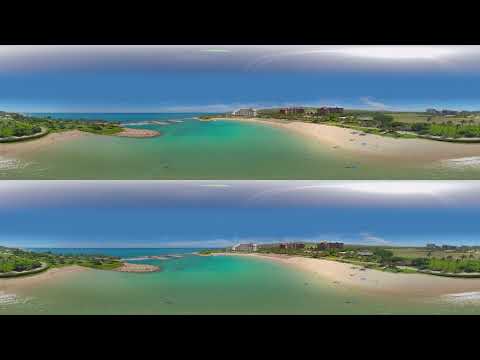The image is a panoramic photograph, duplicated with an identical lower and upper section. The scene showcases a rocky shoreline transitioning to a marshy area that then leads to a beach or a small island, lush with trees varying from small to tall. The vivid blue sky dominates the background, while a brilliant, white explosion of light—likely the Sun illuminating surrounding clouds—sits above the island. The water has receded, revealing a muddy, swirly pattern in the foreground, and the overall aesthetic is natural and serene, embodying a coastal landscape at either sunrise or sunset. There is a vague, superimposed watermark or logo on the left side near the illuminated clouds, adding a subtle layer of texture to the composition.